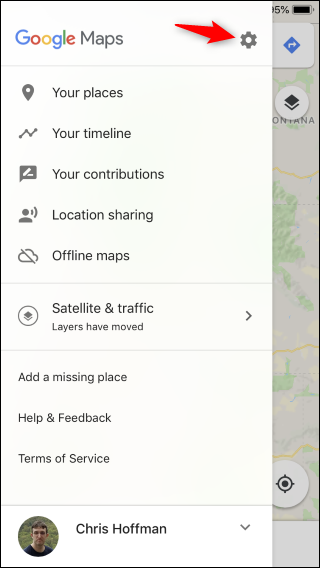This is an annotated screenshot displaying a partially opened tab on the right side, giving the image a somewhat faded appearance in that area. On the top right corner of the screen, there is a black battery bar showing "95%," and further to the right, a search bar featuring a blue diamond with a white arrow is partially visible. Directly below this, fragments of a map with tan, green, and orange elements can be discerned.

On the left side of the image, a thin black border surrounds the contents. The words "Google Maps" are prominently displayed in bold lettering. Adjacent to this text, a thick red arrow points towards a black settings icon. Below this section is a thin gray line, followed by a series of five icons on the left, each accompanied by descriptive text on the right. The first icon resembles a location marker with the text "Your places" next to it, and the second icon, resembling a stock market graph, is labeled "Your timeline." The descriptions of the remaining three icons are not fully detailed.

Another thin gray line separates these icons from an additional icon labeled "Safety and traffic." Below this, there is a notification stating "Layers have moved," accompanied by another gray bar. The bottom portion of the screenshot includes three more lines of information, although their specific contents are not detailed.

In the bottom left corner, there is a small photograph of a man with short brown hair wearing a green shirt, standing against a green backdrop. To the right of the photograph, the name "Chris Hoffman" is displayed.